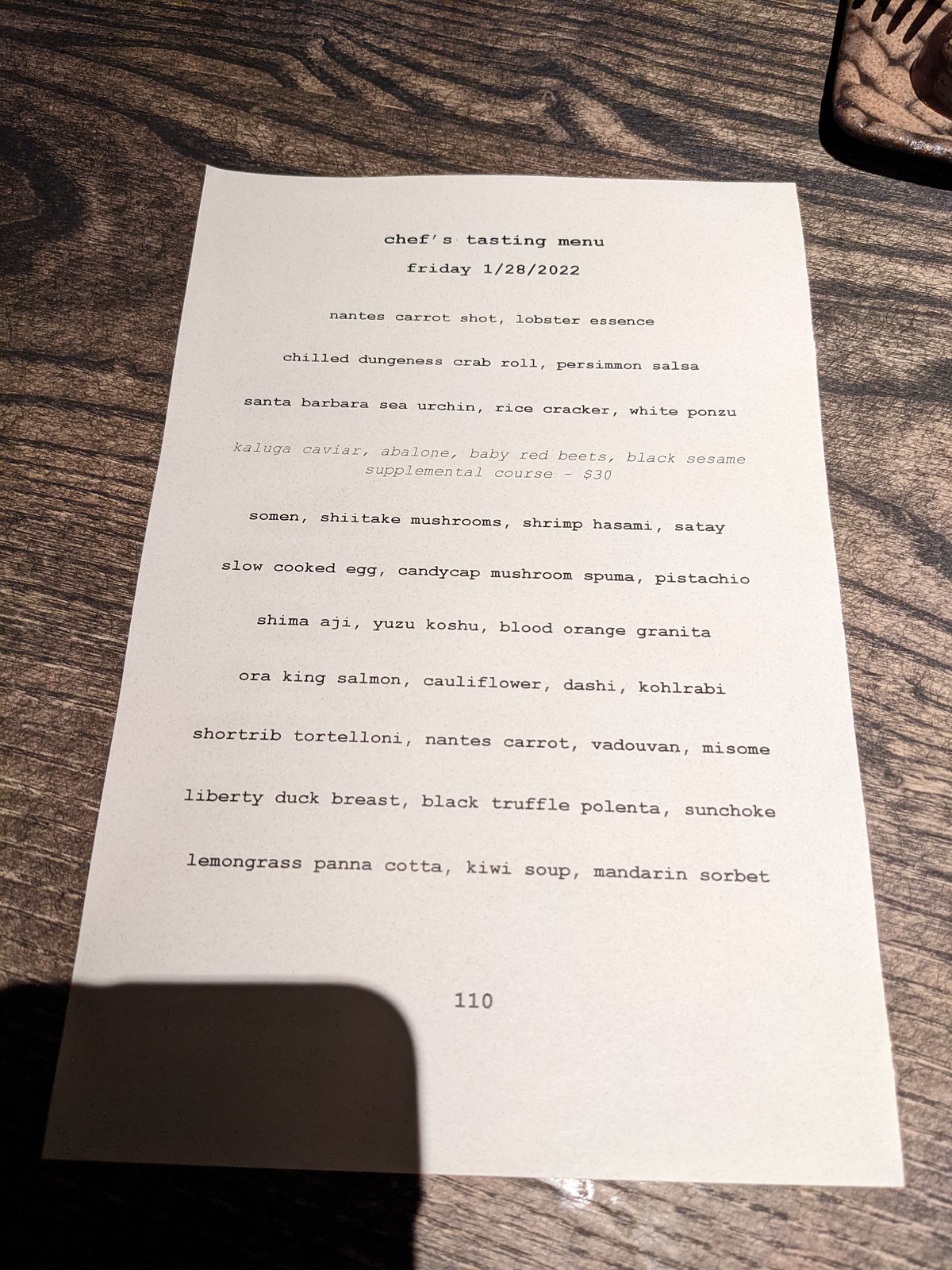A piece of paper rests elegantly on a dark wooden table, displaying a meticulously curated "Chef's Tasting Menu" in black text at the top. Underneath the heading, the date "Friday 1/28/2022" is prominently displayed. The first course listed is "Nantes Carrot Shot, Lobster Essence," followed by "Chilled Dungeness Crab Roll, Persimmon Salsa." The subsequent course features "Santa Barbara Sea Urchin, Rice Cracker, White Ponzu," and the next line details "Kaluga Caviar, Abalone, Baby Red Beets, Black Sesame," with a supplemental course option for $30.

Continuing down the menu, one will find "Somen, Shiitake Mushrooms, Shrimp Hasami, Satay," and "Slow Cooked Egg, Candy Cap Mushroom Spuma, Pistachio." The following course is "Shima Aji, Yuzu Koshu, Blood Orange Granita," followed by "Ora King Salmon, Cauliflower, Dashi, Kohlrabi." The next delicacy listed is "Short Rib Tortelloni, Nantes Carrot, Vadouvan, Miso," succeeded by "Liberty Duck Breast, Black Truffle, Polenta, Sunchoke." The final treat is a "Lemongrass Panna Cotta, Kiwi Soup, Mandarin Sorbet." Centered at the bottom of the page, the price "$110" is clearly printed.